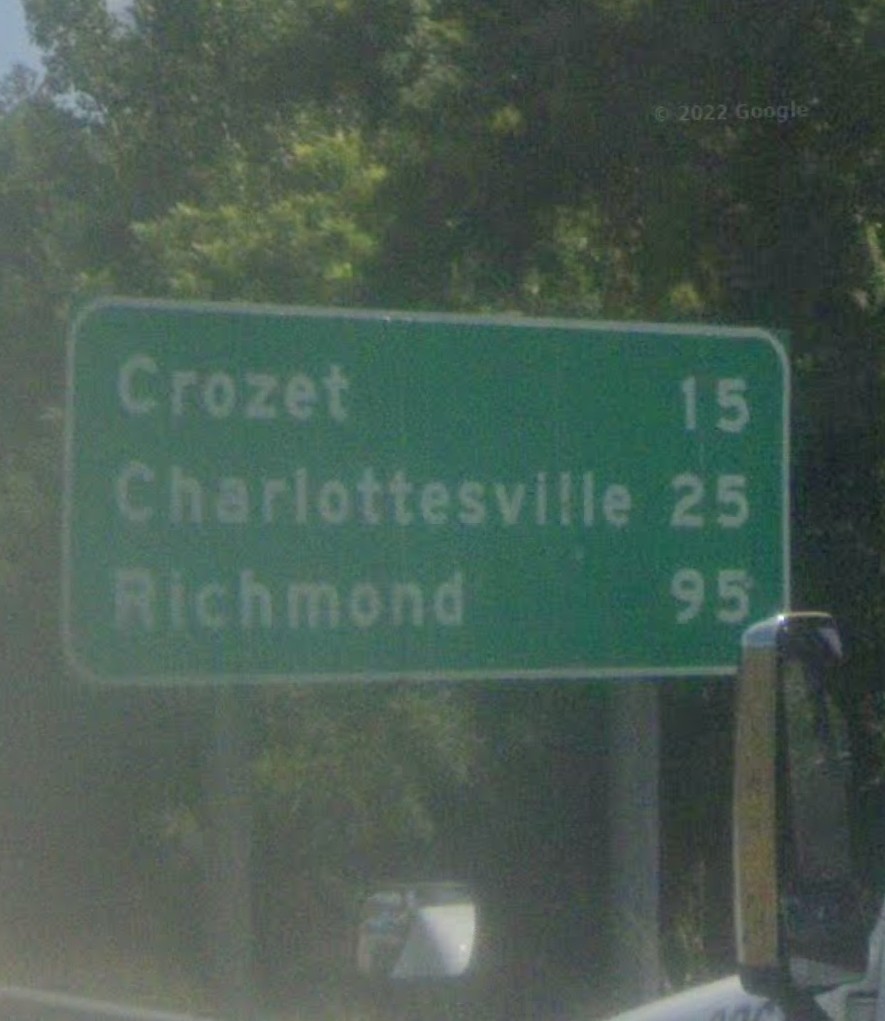A photograph captures the view from inside a vehicle, directing attention to a green roadside sign that details the distances to upcoming towns. The sign indicates that Cosay is 15 miles away, Charlottesville is 25 miles, and Richmond is 95 miles. The sign, standard in design with a green background, white outline, and white lettering, stands prominently amidst a backdrop of lush green trees. Evidence of the vehicle's interior is visible at the bottom of the image, including multiple rearview mirrors and a partial air vent, confirming the perspective from within the car. The scene is bathed in bright daytime sunlight under a clear sky, enhancing the vividness of the surroundings.